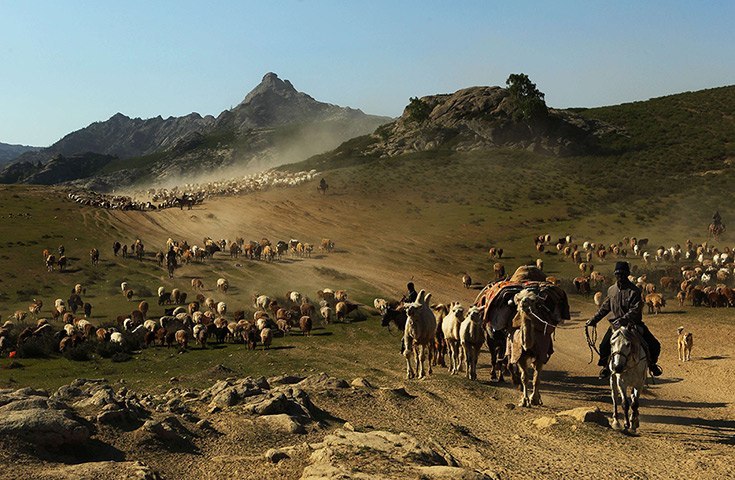In this detailed, somewhat timeless photograph, an organized scene of livestock herding unfolds against a striking backdrop. The focus centers on a trio of horse riders, their figures somewhat indistinct but wearing grayish clothing that blends into the arid, rocky landscape. One horse, notably white, is burdened with various gear. Trailing behind a rider on a white horse is a camel, laden with numerous items. A few other camels linger in the background without any loads.

Scattered around the ensemble are numerous sheep, spread across the area as the herders work to gather them. Amongst the livestock are a couple of dogs, contributing to the herding efforts. The expansive setting features a mixture of green grass and sparse vegetation, with well-worn tracks hinting at the nomadic movements of this group.

The environment is framed by majestic, gray rocky mountains under a vast, clear blue sky free of clouds. This scene, rich in detail yet muted in color, almost resembles a painting with its portrayal of a well-coordinated endeavor to move animals, possibly for grazing purposes. The dusty, immersive atmosphere of this outdoor expedition emphasizes the timeless and enduring nature of the nomadic lifestyle.